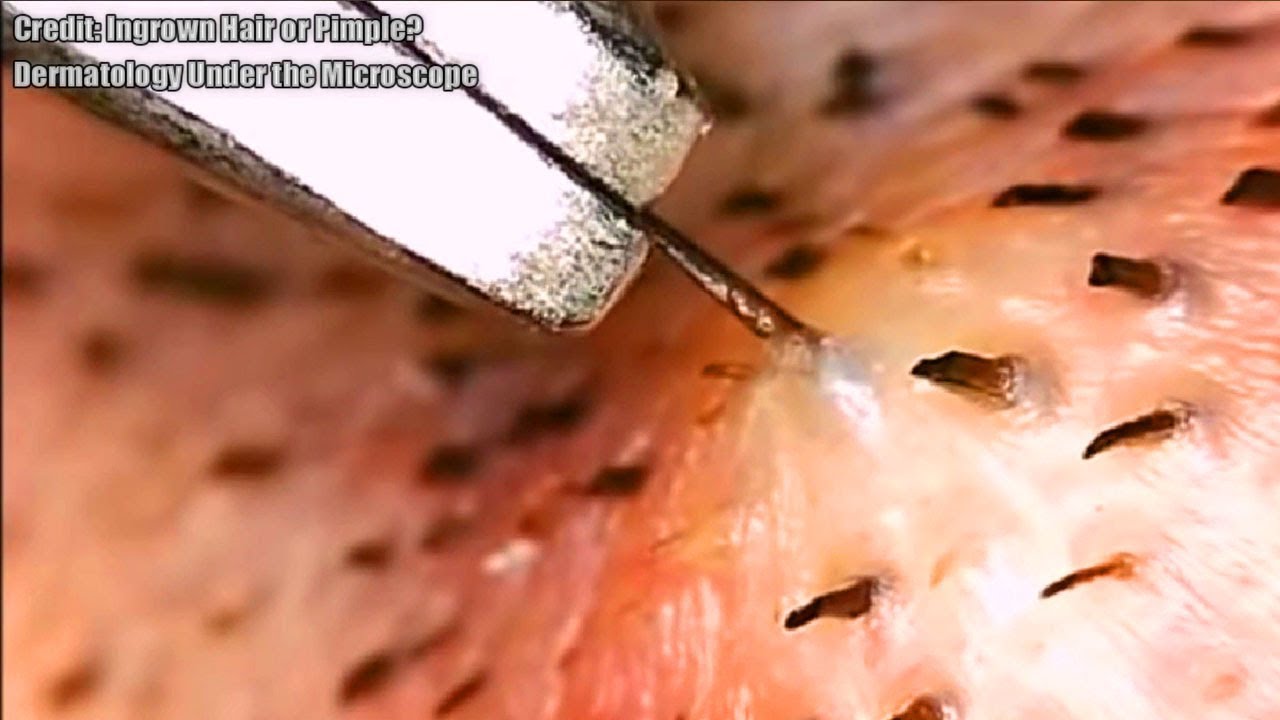The image is a highly-magnified, microscopic photograph of a section of Caucasian skin, showcasing its pinkish, slightly oily surface dotted with sparsely spaced, black hairs. Among these hairs, one is prominently being gripped by the shiny, metal ends of a pair of tweezers, which are exerting a pull on the hair, causing the skin to strain subtly at the root. Each hair follicle appears jagged at the ends with swollen roots embedded in the skin, reminiscent of pin feathers on chicken skin. In the upper left corner of the image, text in white font with a black outline reads, "credit: ingrown hair or pimple?" followed by a new line stating, "Dermatology under the microscope."